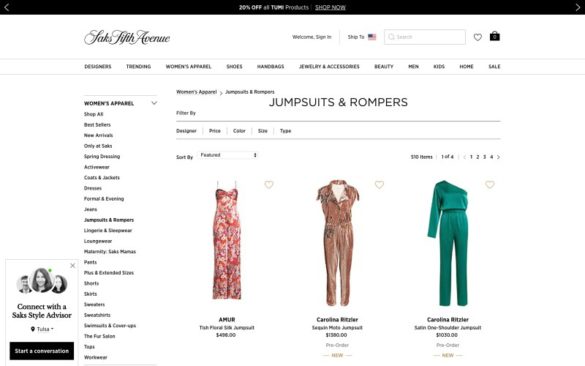This image is a screenshot of a Saks Fifth Avenue webpage, characterized by its clean white background. At the top, there's a thin, gray to black upper banner. Indented slightly from the left-hand side, a vertical drop-down menu appears against the white background, accompanied by a small advertisement in the lower left-hand corner inviting users to "Connect with a Saks Style Advisor," including a "Start a Conversation" button.

At the top of the menu, the women's apparel section is prominently displayed with a dropdown arrow for more options. Directly below this, the "Jumpsuits" category is listed. Adjacent to the Saks Fifth Avenue logo on the top banner, options such as "Welcome," "Sign In," a search bar, a flag icon, a heart icon, and a shopping bag icon are visible, allowing easy navigation.

The main page headline, "Jumpsuits and Rompers," is centered at the upper part of the screen, with various filter options underneath, including designer, price, color, size, and type. Featured products are displayed prominently.

Three outfits are showcased horizontally from left to right: a pink floral strapless dress, a short-sleeved terry brown jumpsuit, and a long-sleeved green jumpsuit.